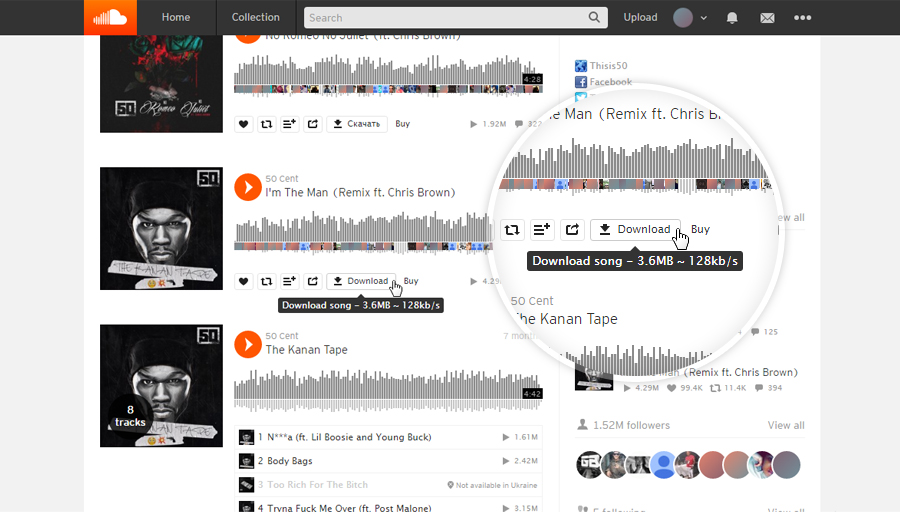The image showcases the SoundCloud website interface. At the top left corner, the iconic SoundCloud logo is prominently displayed, featuring a distinctive orange box with a cloud, half of which incorporates sound bars. The top navigation bar includes several essential tabs: 'Home,' 'Collection,' 'Search,' 'Upload,' 'Account,' along with a bell icon for notifications and a mail icon for messages.

The screen is focused on sound media files by the artist 50 Cent, highlighting two specific tracks. The first prominent track in the middle is "I'm the Man (Remix)" featuring Chris Brown. An orange play button is visible next to the track, signifying it can be played directly. Currently, the user's mouse cursor is hovering over the 'Download' option for this song, indicating an attempt to download the 3.6-megabyte file. Below this track is another by 50 Cent titled "The K9 Tap Tape." To the right side of the screen, there is a magnified view of the mouse pointer, clearly emphasizing the user's intent to download "I'm the Man (Remix)."